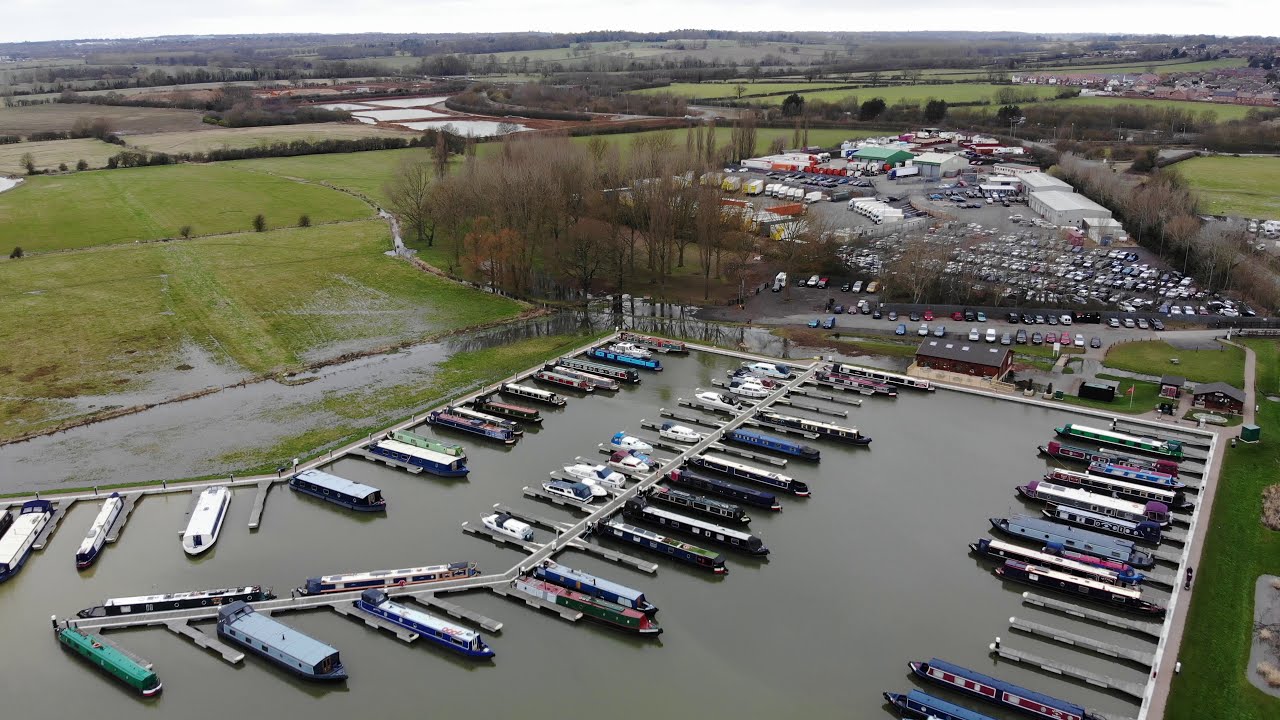This image depicts an aerial view looking down on an intricately sectioned-off, rectangular boat dock. The dock is split down the middle, creating two lengthy rows with boats docked on either side, resulting in four distinct parking lanes. A kaleidoscope of colors is seen among the boats, with notable mentions including dark and light green, maroon and black, blue, purple, blue and white, light grey, yellow, red, and combinations of red and white. Surrounding the dock, the scene expands into a variety of landscapes, featuring a wet grassy perimeter, numerous trees, and bushes. To the upper right, there is a secondary parking lot filled with cars and further bordered by scattered buildings, possibly businesses, all set within a vast open field.